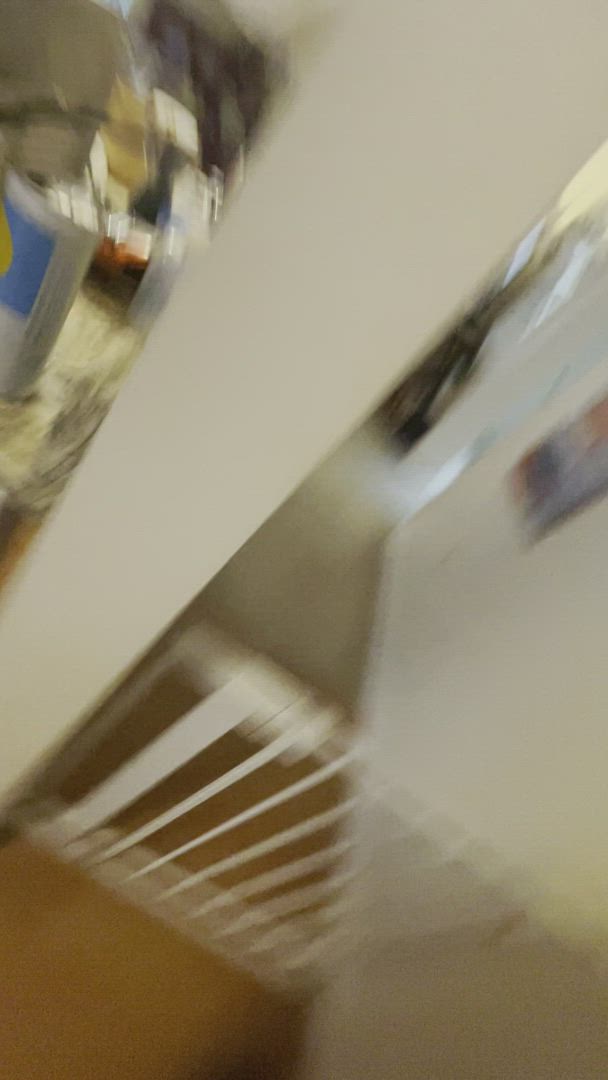A slightly blurred photograph captures a transitional moment during a move, focusing on the entrance to a hallway. The image is taken from what appears to be the kitchen area, evidenced by a cluttered countertop to the left piled with moving boxes and a small canister, likely for seasoning. A baby gate sections off the hallway, suggesting that this area leads further into the house. Despite the motion blur, it is clear that the space is mid-transition, reflecting the activity of packing and preparing for relocation.